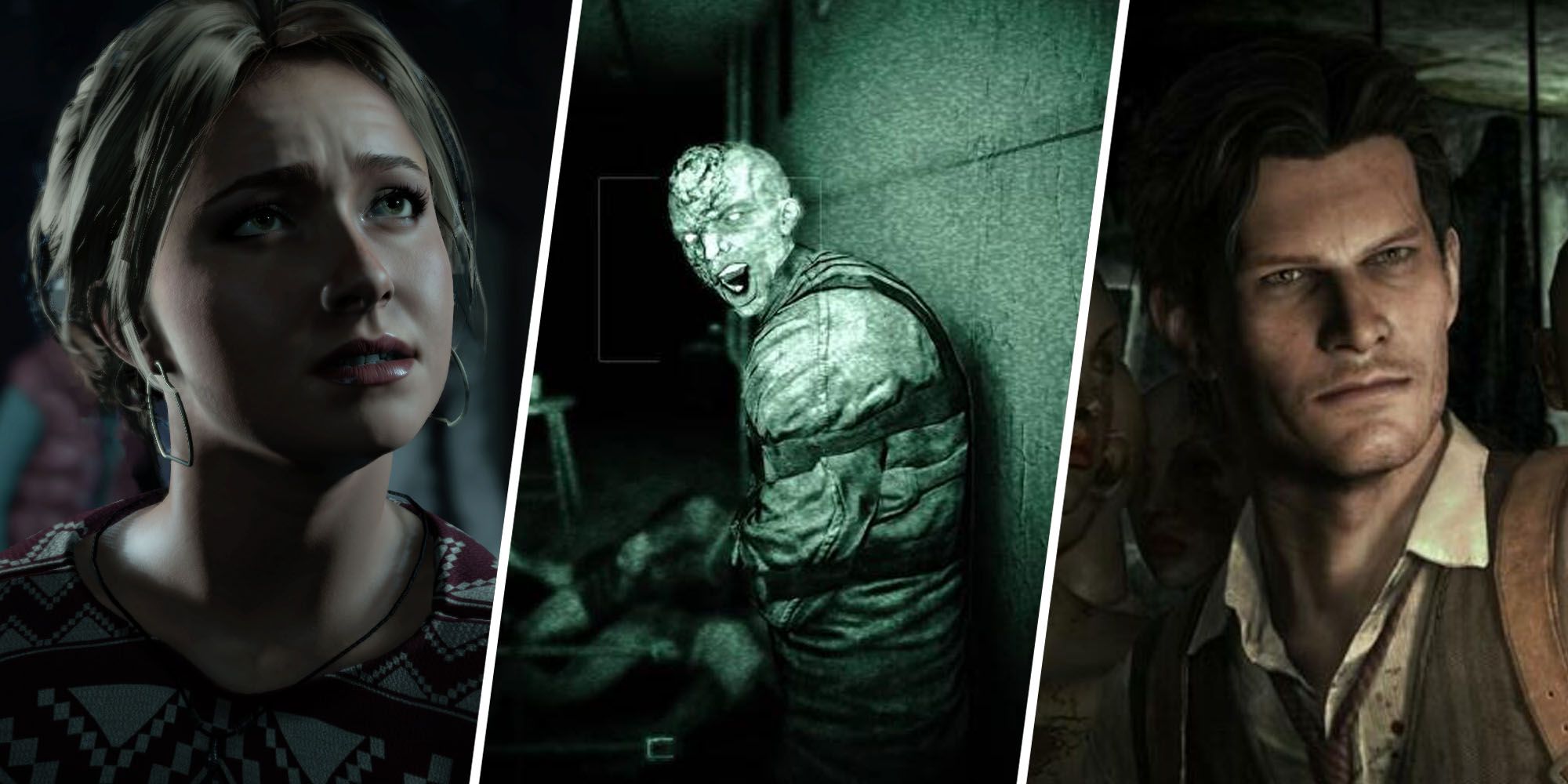This is a horizontal rectangular image divided into three vertical segments by white lines. Each segment showcases a different character, seemingly from a video game or a movie titled "Until Dawn." 

On the left side, there's a realistic-looking woman with blonde hair that falls slightly below her ears. She has earrings, a round-collared shirt with a red and white graphic design, and a necklace. Her expression is one of concern as she gazes slightly to the right and up.

The middle segment features a CGI or animated monster with a pale, almost white head, and a body strapped with what appears to be a straitjacket. The monster's head is turned back and it appears to be screaming, with a blurry gray wall and possibly dead or injured people in the background.

The right segment shows an animated man with medium-length brown hair. He wears a light-colored collared shirt under a brown or gray vest, complemented by a brown jacket. His body is slightly turned to the left, and part of a potentially gun-like object is seen over his shoulder. The dark background here makes other details indistinguishable.